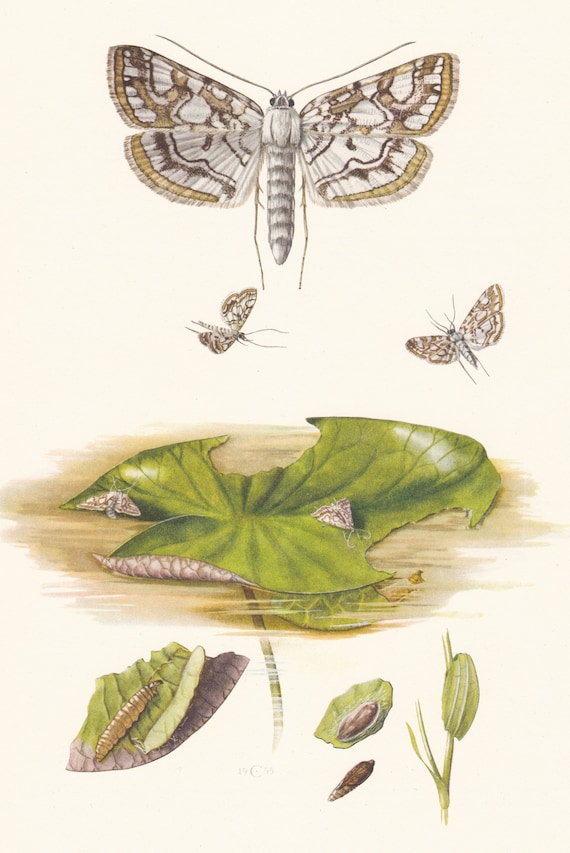This illustration features a meticulously drawn and colored depiction of various stages of moths and butterflies, centered around a large, dominant moth with its wings spread wide. The colors of the central moth are a blend of light gray, light yellow, and dark brown. Below this central moth, two smaller moths or butterflies are in flight, adding to the sense of movement across the image. The background is a light brown, creating a warm and cohesive backdrop for the scene.

In the lower part of the image, a green, chewed-up leaf hosts two tiny moths. The leaf has noticeable chunks missing from its corners, indicating it has been nibbled on. Scattered beneath this leaf are leaf fragments and larvae, illustrating the metamorphosis process from caterpillar to moth. This visual narrative mirrors how a butterfly transitions from caterpillar form, suggesting these are the earlier stages before becoming the large moth featured at the center.

In addition to the intricate details of the moths and their life stages, there is a small inscription at the bottom center of the image reading '19C55' or possibly 'SS,' which may reference the artist or the piece's creation date. The illustration masterfully combines natural elements and detailed artistry to depict the lifecycle of moths and butterflies.